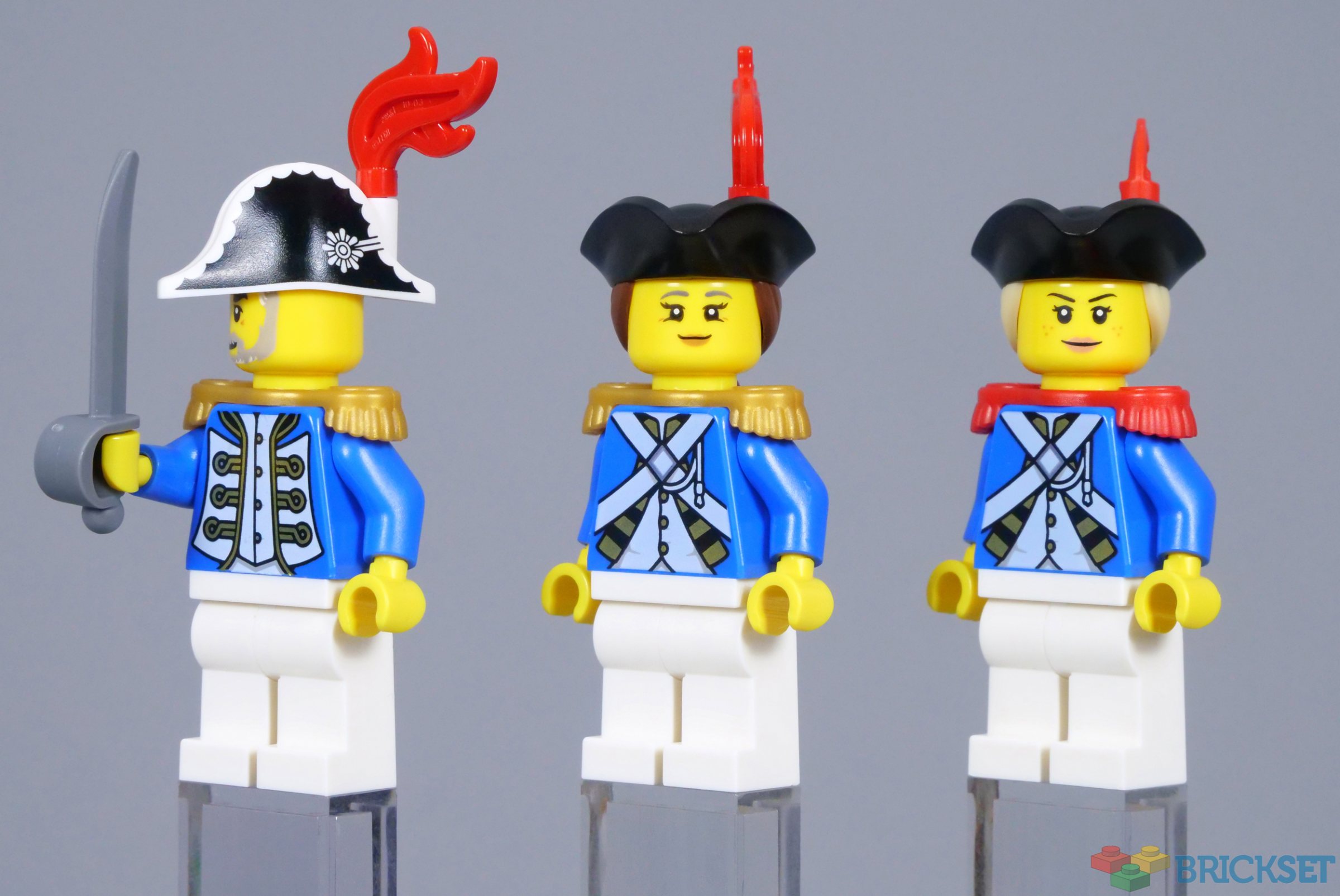The image features three Lego figures positioned against a bluish backdrop, labeled "Brick Set" in the bottom right corner. These figures resemble military characters, each adorned with distinctive uniforms and accessories.

Starting from the left, the first figure is a male character with a black and white admiral's hat, featuring a red feather-like flame protruding from the top. He has a silver beard and sideburns and is dressed in a blue vest with golden and white detailing, paired with white pants. This character carries a silver sword in his right hand and sports golden fringe on his shoulders.

The central figure is a female character, similar in attire to the first, wearing a blue shirt with white pants. She has an all-black three-pointed hat, also decorated with a red flame. She features brown hair and golden shoulder pads, adding a touch of distinction from the other figures.

On the far right is another female figure, mirroring the outfit style of the other two with a blue shirt and white pants but with red shoulder pads instead of gold. She wears the same black hat with a red flame and has blonde hair.

All three Lego figures share yellow-colored hands and faces, and they stand on silver spike-like bases, enhancing their military appearance.